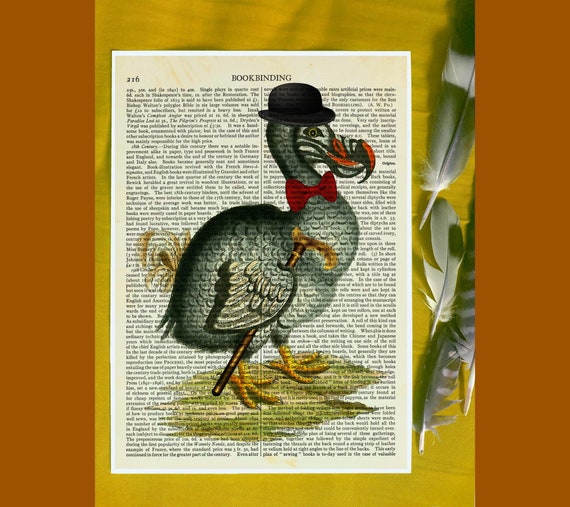This image captures a page from a book set against an orange background with a yellow overlay in the center. The page features two columns of black text, with the number "216" at the top and the words "book binding" prominently displayed in the middle. Superimposed on this page is an illustration of a duck wearing a black bowler hat. The duck, depicted in shades of blue and gray, sports a red bow tie and yellow feet. It holds a brown cane with a yellow or gold handle. Additionally, several feathers are scattered to the right side of the page, extending beyond its edges.